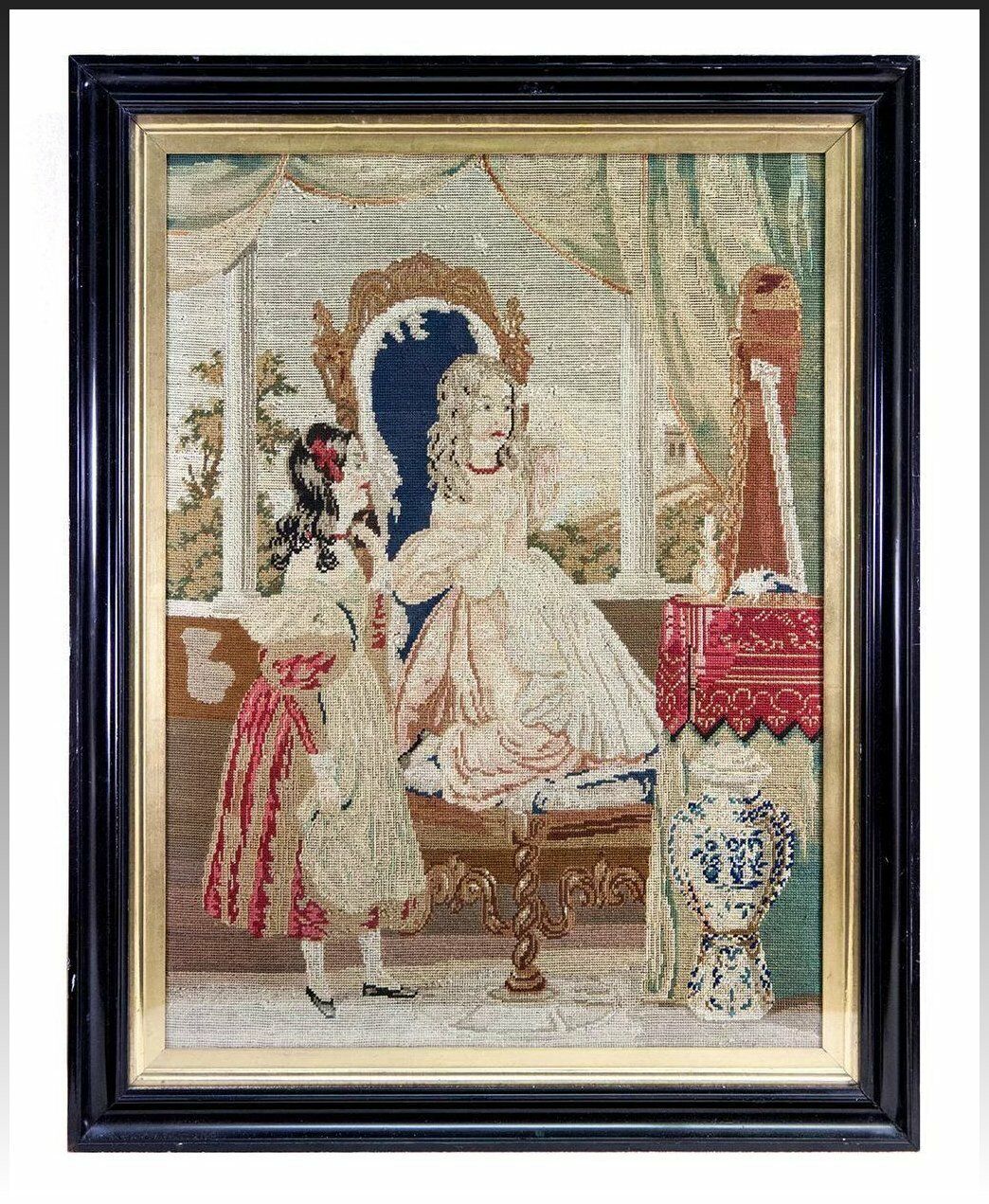This detailed Victorian needlepoint tapestry, framed with a matte black outer frame and an inner gold trim, portrays a scene of elegant opulence and artistry. It captures two girls inside a lavish room with an open window behind them, revealing a lush outdoor setting with trees and plants seen through billowy green and cream drapes. 

The central figure sits on a very stylized, ornate golden chair with a blue back and white border, indicating her high status. She has blonde hair and wears a long pink and white ruffly dress. This girl gazes into a mirror on a red-clothed vanity in front of her. Standing beside her is a girl with dark hair adorned with a red barrette or headband with red flowers. She wears an off-the-shoulder dress in hues of red and brown, accentuated with a white apron-like front and leg-of-mutton sleeves, and black shoes.

On the floor near the vanity rests a beautifully detailed blue and white urn, enhancing the room's richness. The surrounding elements, including the meticulous stitching details and faded hues of the tapestry, emphasize the craftsmanship and historical essence of the piece. This handcrafted work reflects the elegance and wealth of the depicted time period, making it a striking and evocative piece of art.